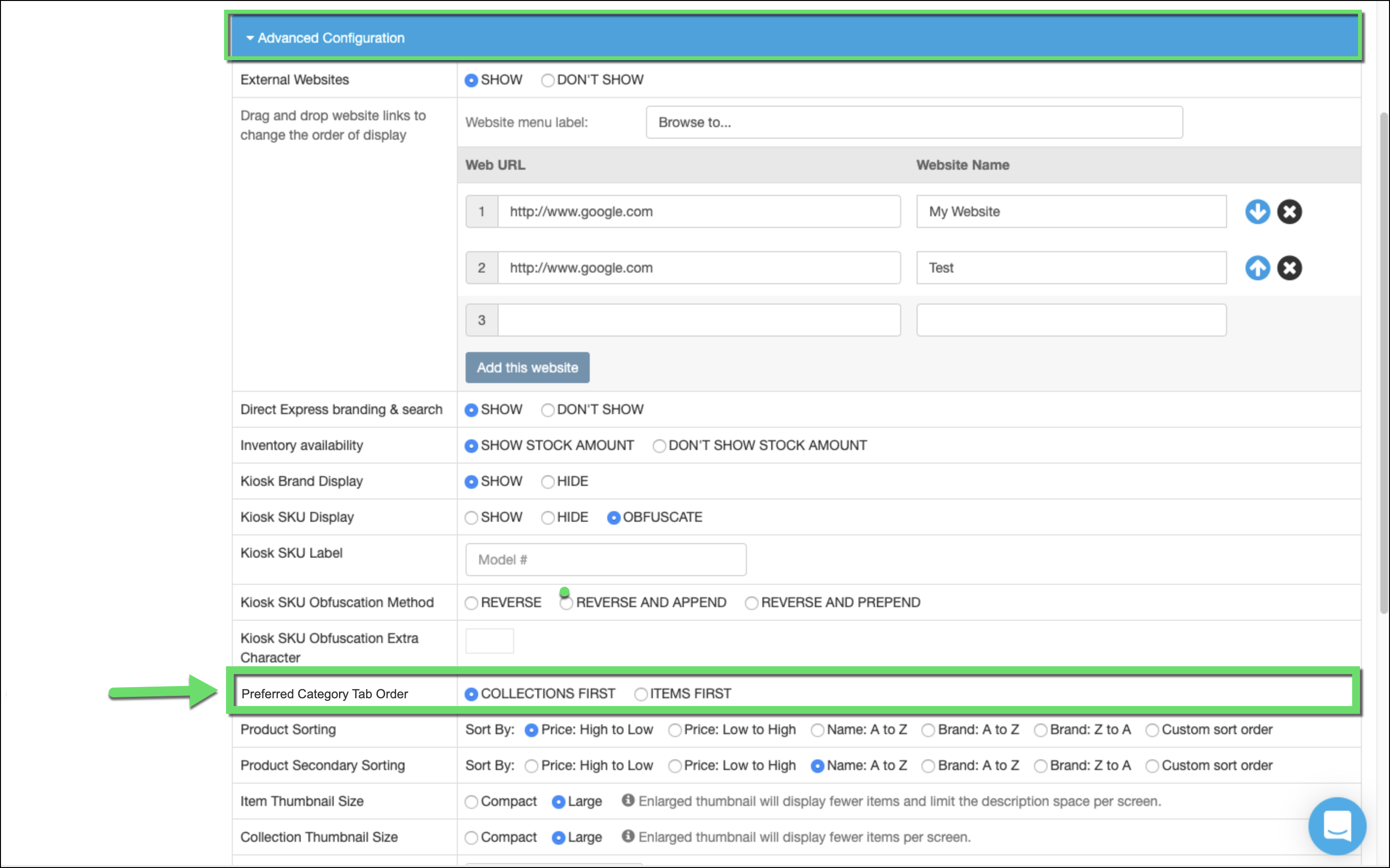The image depicts a detailed screenshot of a desktop interface, most likely from a website or software dedicated to setting up an online shopping platform. At the top of the interface, a green highlighted area indicates the current active category, suggesting instructional context.

Centered in a blue rectangle with white text, the heading reads "Advanced Configuration." The interface displays a chart organized into several configurable sections, guiding users through intricate setup options for an e-commerce site.

From left to right, the chart includes the following configuration options:
1. **External Websites:**
   - "Show," "Don't Show," or "Show as Toggled"
   - Functionality to drag and drop website links to reorder their display
   - Fields labeled "Website Menu Label" and "Browse to..." for customizing the link text and directing to specific URLs
   - Options for Web URL versus Website Name.
   - Example Entries: "Google's website" labeled as "My Website" and "Google" labeled as “Test”

2. **Direct Express Branding and Search:**
   - Options: "Show," "Don't Show," or "Show as Toggled"
  
3. **Inventory Availability:**
   - Toggle to "Show Stock Amount" or "Don't Show Stock Amount."
  
4. **Kiosk Brand Display:**
   - Options to "Show as Toggled" or "Hide"
  
5. **Kiosk SKU Display:**
   - Options: "Show," "Hide," or "Obfuscate" (the latter implying to hide or confuse the visibility of SKU numbers)
   - A text box labeled "Kiosk SKU Label," likely for entering SKU or model numbers.

6. **Kiosk SKU Obfuscation Method:**
   - Options to "Reverse," "Reverse and Append," or "Reverse and Prepend" the SKU number, with "Reverse and Append" being highlighted by a green dot as the selected method.
   - Text box labeled "Kiosk SKU Obfuscation Extra Character" positioned beneath a prominent green rectangle with an arrow.

7. **Preferred Category Tab Order:**
   - Options: "Collections first" (selected) and "Items first."
  
8. **Product Sorting:**
   - Primary sorting options: "Price high to low," "Price low to high," "Name A to Z," "Brand A to Z," "Brand Z to A," and "Custom Sort Order," with "Price high to low" currently selected.
   - Secondary sorting options with similar choices, currently showing "Name A to Z" as selected.

9. **Item Thumbnail Size:**
   - Options: "Compact" or "Large," with "Large" selected.
   - Note indicating that larger thumbnails will display fewer items and reduce description space per screen.

10. **Collection Thumbnail Size:**
    - Options: "Compact" or "Large," with "Large" selected.
    - Note indicating that larger thumbnail sizes will display fewer items per screen.

In summary, the image showcases a meticulous setup interface for configuring various aspects of an online shopping site, including website links, inventory display, kiosk settings, category arrangement, product sorting, and thumbnail sizes.